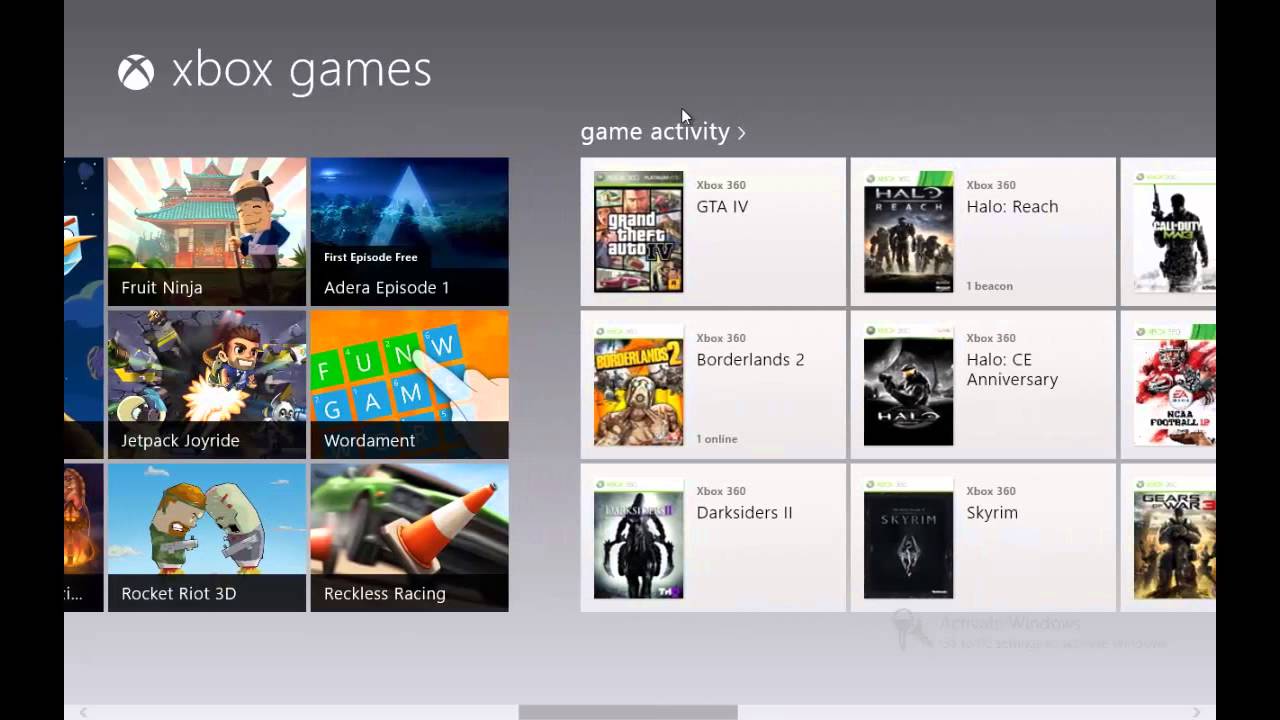This image depicts a screenshot taken in landscape mode during the process of scrolling through a website by the creator. Evident from the middle of the image, a black stripe vertically divides the screen, indicating active scrolling from top-left to bottom-left and top-right to bottom-right. Partial images are visible on both sides of the stripe, reflecting the incomplete transition between content sections.

In the upper left corner, the text "Xbox games" is displayed, introducing a collection of game titles featured on the site. The showcased games, "Fruit Ninja," "Adira Episode 1," "Jetpack Joyride," "Wordament," "Rocket Riot 3D," and "Reckless Racing," are organized in a grid of three rows and two columns.

Adjacent to this game list, on the right side, the heading "Game Activity" accompanied by a right arrow is visible. This section appears to highlight recent activities or games played, possibly by the user or their friends, including titles such as "Grand Theft Auto," "Halo Reach," "Halo CE Anniversary," "Borderlands," "Darksiders," and "Skyrim." The presentation of this activity suggests tracking of recent gameplay, likely indicating the games currently or recently played by the user or their friends.